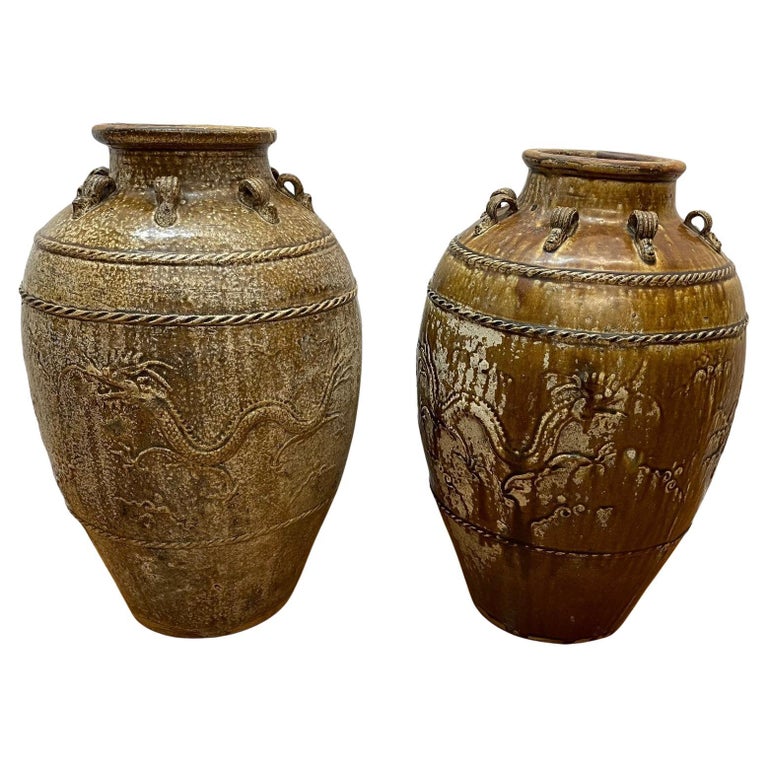The image features two vases set against a white background, giving the impression that they are floating in space. Both vases are made of a dark, shiny material—possibly metal or ceramic—and exhibit a weathered, antique appearance with a predominant brownish color, accented by lighter, off-white patches. The vase on the left is slightly larger than the one on the right. Each vase is adorned with intricately carved designs, including coiled rope-like adornments around the neck and base, and elaborate dragon motifs. The dragons, depicted in a style reminiscent of oriental art, feature serpentine bodies that wrap around the vases, with tails and heads clearly visible. Despite the carvings, there are no protruding elements; all designs are indented into the vase surface. This craftsman work creates an impression of ancient, utilitarian jars that may have once been used for carrying water.